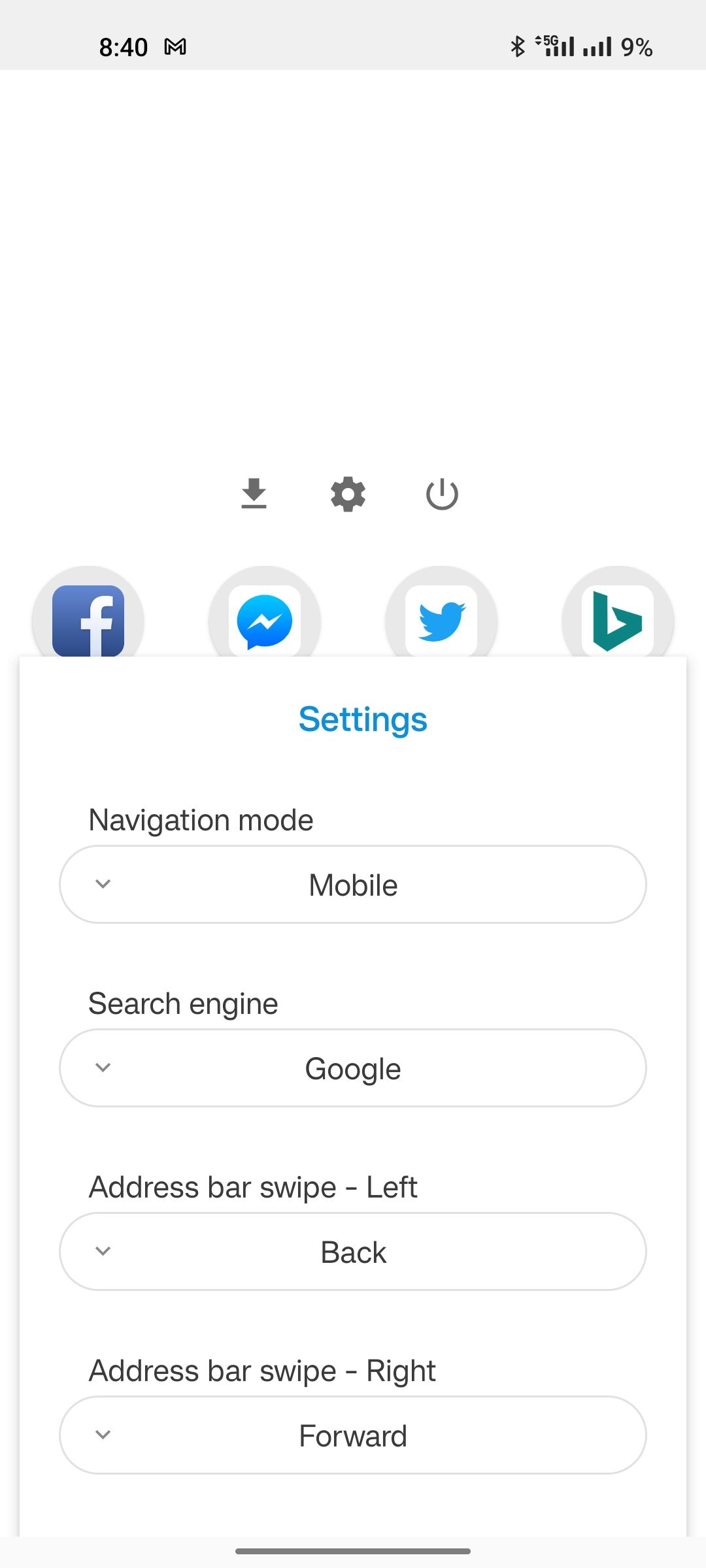This is a detailed screenshot of a mobile phone's display showing a pop-up settings menu at the center. At the top of the screen, a light gray header bar provides basic phone and carrier information. The left corner shows the time as 8:40 AM. Adjacent to the time is the carrier's logo, an outline of the letter "M" resembling bubble art with an unfilled center. 

To the right side of the header, several icons are visible: a Bluetooth symbol, a 5G signal strength indicator with five ascending bars, a cellular service signal indicator with four bars, and a battery icon displaying 9% charge.

Beneath the header is a white space area with three centered buttons. From left to right, the icons represent "Download," "Settings," and "Power." Below this button trio is a row of four app icons: Facebook, Messenger, Twitter, and what appears to be the Microsoft Store, symbolized by a script-styled triangle with an open top.

The main focus of the screenshot is the white pop-up settings menu with slightly grayed sides and a faint shadow giving it a three-dimensional effect. The heading "Settings" is displayed in light blue text. The menu contains four drop-down options each outlined in a thin gray line with white fill and a drop-down arrow on the left. These options are:

1. **Navigation Mode:** Displays "Mobile" in the center.
2. **Search Engine:** Displays "Google" in the center.
3. **Address Bar Swipe Left:** Displays "Address Bar Swipe Left" in black text.
4. **Address Bar Swipe Right:** Displays "Forward."

At the bottom of the screenshot, there is a dark gray horizontal line, centered and encompassing about one-third of the phone's width.